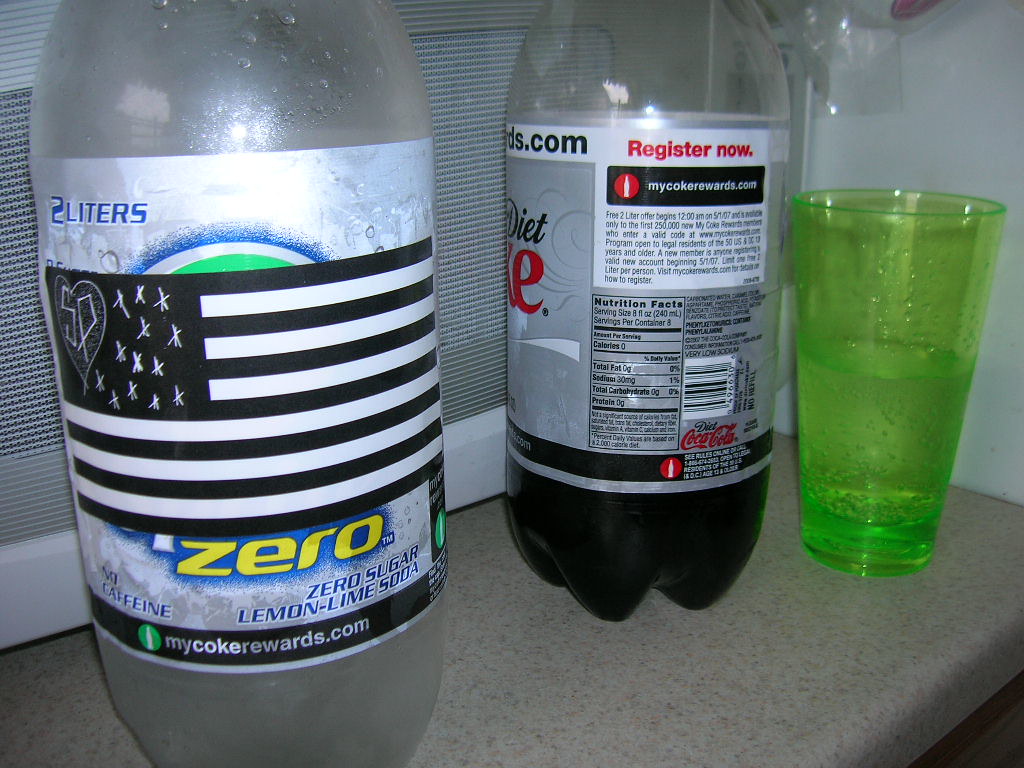The image captures two 2-liter bottles prominently positioned on a sideboard in a kitchen setting. The photo is taken from a lower left angle, extending towards the upper right, which gives a dynamic perspective. One of the bottles appears to be a soft drink labeled "Zero" and features a black and white American flag motif on its label, evoking a patriotic theme. The adjacent bottle is a recognizable Diet Coke. Behind the bottles, there is a microwave door visible, adding context to the kitchen environment. The front edge of the sideboard and a portion of a cabinet on the lower right are also in view, enhancing the sense of depth in the room. To the far right of the frame, a green cup is placed, adding a pop of color to the scene.